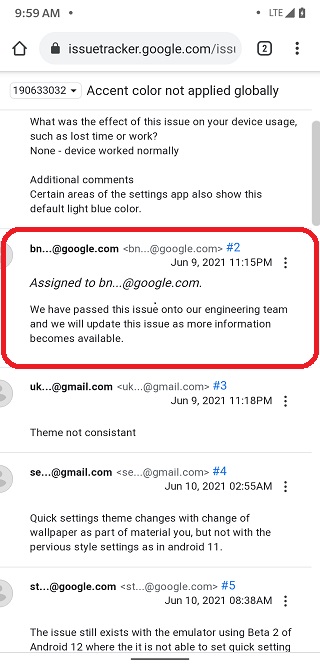This is a detailed, descriptive caption for the given image:

---

The screenshot captures a mobile device displaying an email browser, possibly the Google Chrome app. In the upper left corner, the screen shows the current time as 9:59 a.m. with a small dot next to it. On the upper right, there is another dot followed by "LTE," a signal triangle icon, and a battery icon indicating the device is charging—all icons are in dark gray against a light gray or white background.

Beneath this status bar, the browser navigation row appears. On the far left, there's a home icon. Just right of center is the URL bar containing a padlock icon, with the text "issuetracker.google.com/issi…" truncated. To the right of the URL bar, a small square containing the number 2 indicates multiple open tabs. Next to this is a three-dot menu icon.

The primary content of the screenshot starts below this navigation row, showing what looks like an email chain or conversation. At the top is a rectangular box with a light gray border containing the number "1906333032" and a downward-pointing arrow. Adjacent to this, in uppercase text, is "Accent color not applied globally."

The main content contains a series of questions and responses likely part of an issue report. Questions such as "What was the effect of the issue on your device usage such as lost time or work?" followed by the response "None, device worked normally” are visible. Additional comments note, "Certain areas of the settings app also show this default light blue color."

Further down, details resembling individual emails begin. Each email starts with an avatar circle to the left, followed by partial email addresses like "BN...@google.com" in light gray, message numbers in blue, and timestamps such as "June 9th, 2021, 11:15 p.m." These emails include messages like "We passed the issue on to our engineer team and we will update this issue as more information becomes available."

The most prominent email has a red curved border outline, highlighting it. Below this highlighted message, there are three more similar email previews, each containing the same structure of avatar, email, text, and timestamp.

This screenshot effectively captures the layout and content of an issue tracker page viewed on a mobile browser.

---